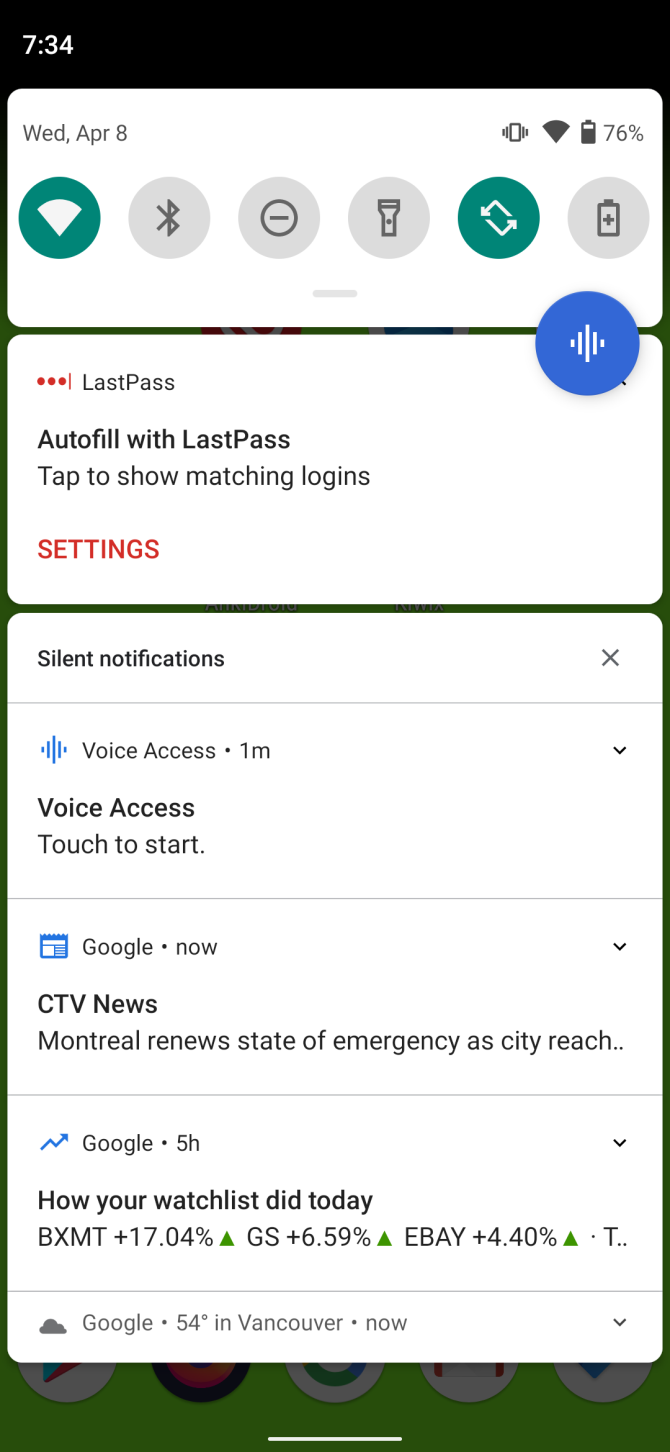Screenshot of an Android phone in portrait orientation. The time is displayed in the upper left corner showing 7:34, without an AM or PM indicator. Below the time is a card displaying "WED, APR 8," signifying Wednesday, April 8th. A vibration icon, which appears unselected or disabled, is displayed next to it. The status bar shows a fully filled Wi-Fi symbol and a battery icon that is three-quarters full, indicating 76% charge.

In the quick settings menu below, there are various icons including Wi-Fi, Bluetooth, a horizontal line with a circle around it (likely Do Not Disturb), a flashlight icon, a rotation lock icon, and another battery icon. Additionally, there is a unique icon with horizontal lines of varying lengths centered by a vertical line, possibly a feature to activate different commands or access.

There are several notification cards below this. One card is for LastPass, followed by a silent notification section. Multiple rows show notifications from apps like Voice Access and Google, listed repeatedly indicating several interactions or updates from these services.